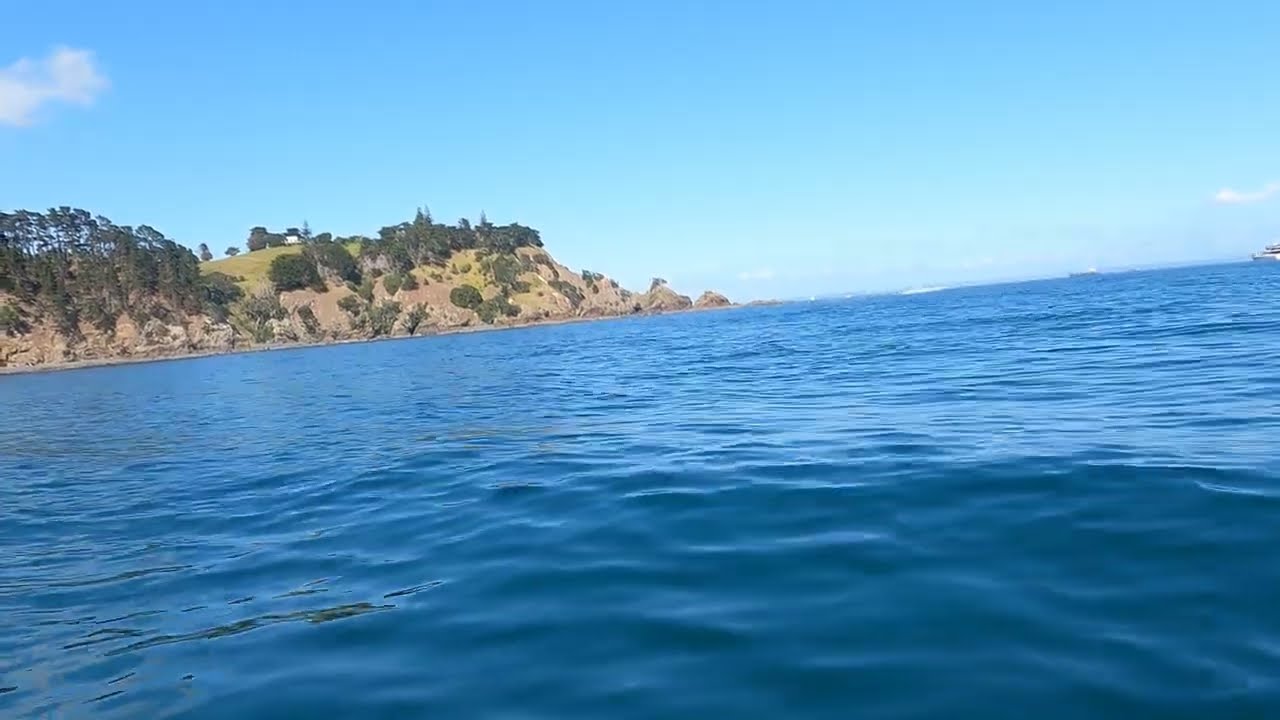The photograph showcases a tranquil ocean under a clear, blue daytime sky with a few scattered clouds. The calm waters, displaying gentle waves and various shades of blue, meet a rugged shoreline on the left side of the frame. This shoreline consists of a rocky formation that ascends gradually from the center, reaches a peak near the top left, and then slopes down slightly, finally ascending again in the extreme left corner. The cliffside is densely adorned with leafy, bushy trees and a well-hidden grove, creating a lush greenery. Near the top of this landform, a small white house with a black roof is perched, adding a quaint touch to the natural scenery. In the background, a large boat is faintly visible near the top right horizon, adding context to the vast expanse of the ocean. The entire scene exudes a serene and picturesque quality, capturing the beauty of nature seamlessly integrated with a touch of human presence.